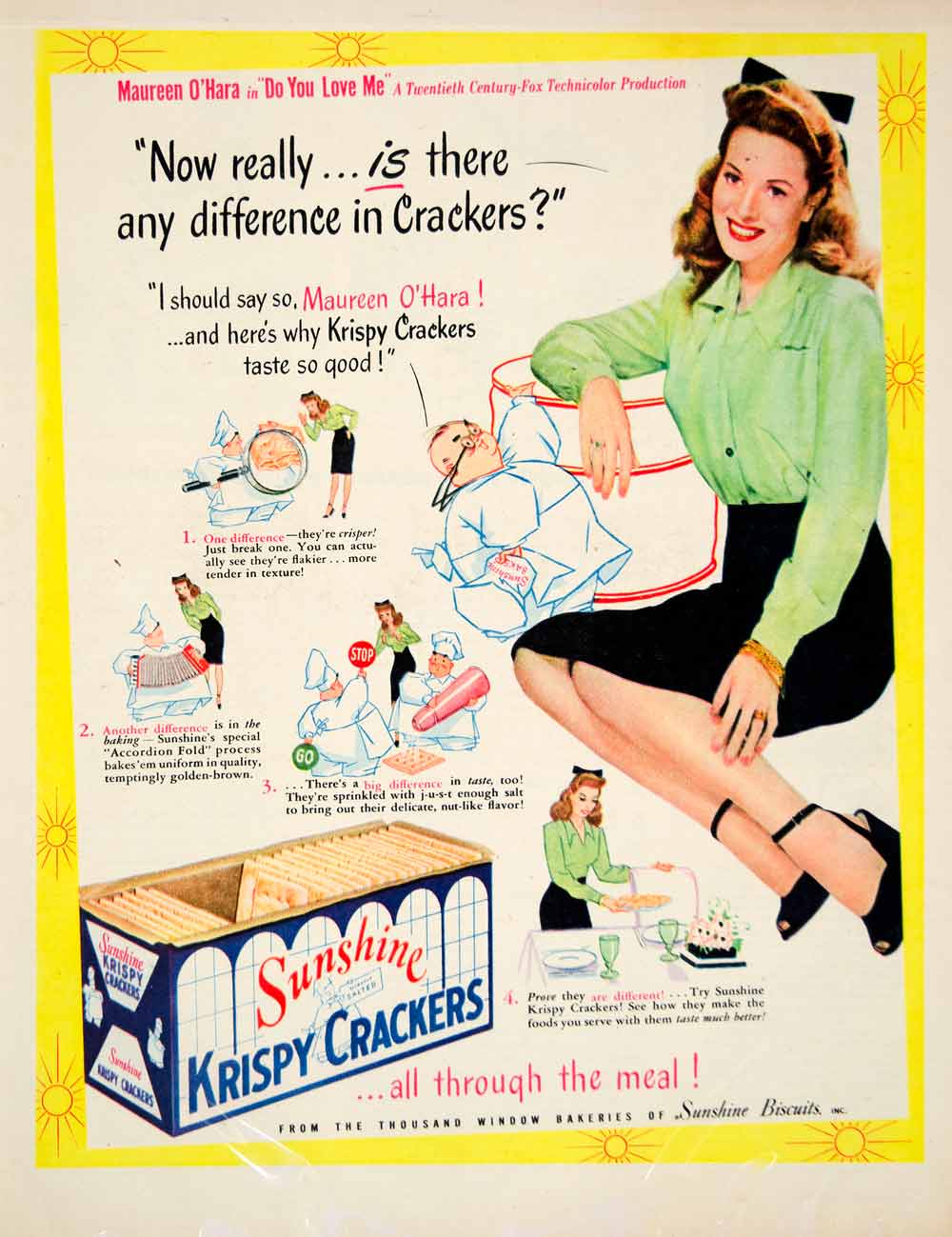This vintage advertisement features the renowned actress Maureen O'Hara, dressed in a sophisticated green button-up shirt with a collar, a long black pencil skirt, and black heeled sandals with straps. Her auburn hair is elegantly styled with a black bow, cascading down her back, emphasizing her classic beauty. The ad prominently displays the title "Maureen O'Hara, Do You Love Me? A 20th Century Fox Technicolor Production" at the top. It underscores the superiority of "Sunshine Crispy Crackers" with bold text reading, "Now really is there any difference in crackers? I should say so, Maureen O'Hara, and here's why crispy crackers taste so good." The ad lists the distinctive qualities of these crackers: their crispier, flakier texture, achieved through a special accordion fold baking process that ensures uniform quality and a tempting golden brown color. It also highlights their delightful nut-like flavor, enhanced by a perfect sprinkling of salt. At the bottom, it encourages readers to "Prove they are different – try Sunshine Crispy Crackers" and see how they enhance the taste of the meals they accompany. The ad is completed with the phrase "All through the meal from the thousand window bakeries of Sunshine Biscuits" and showcases a package of the Sunshine Crispy Crackers on the side, enticing viewers with the image of the golden, flaky saltine crackers inside.